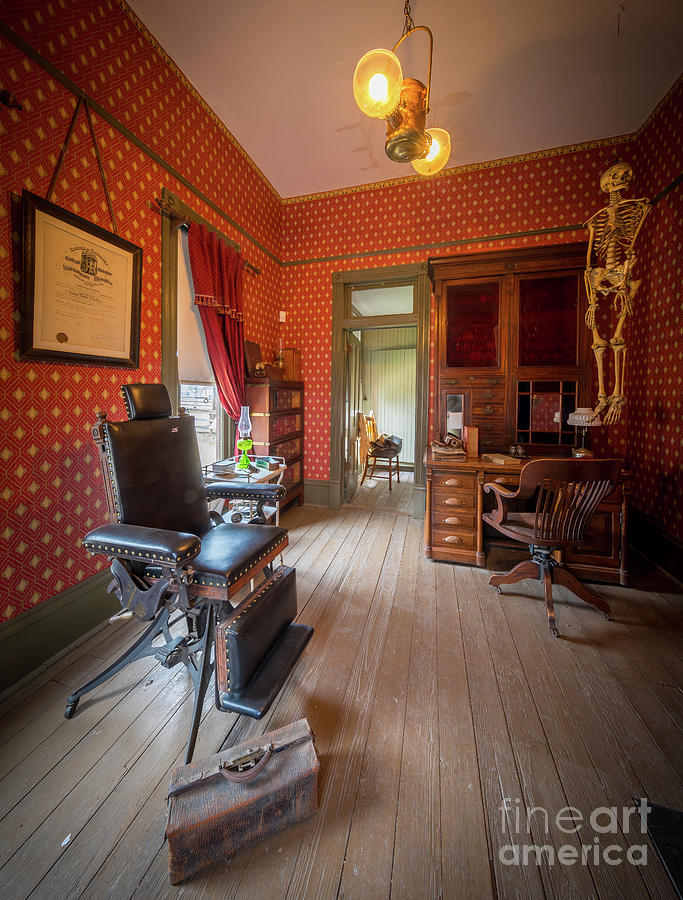This wide-angle photograph captures the interior of a vintage room, likely an old barber's studio or a medical-themed space, showcasing rich historic details. The room features maroon wallpaper adorned with gold patterns, adding a luxurious yet antique feel. The flooring consists of light wooden planks, complementing the vintage ambiance.

Central to the room is a meticulously detailed dark brown leather chair, potentially a barber or dentist's chair, characterized by its metal studs, cushioned leather arms, and a footrest, all supported by sturdy metal legs. Adjacent to this chair is a weathered leather satchel, enhancing the nostalgic atmosphere.

In the right corner, an upright medical teaching skeleton is positioned atop a wooden desk, which boasts numerous pigeonholes and compartments reflective of an old highboy desk. An accompanying wooden chair is pulled up to this desk. The desk itself holds a glass lamp and various pieces of memorabilia.

Further details include a diploma on the wall, red curtains, and a kerosene lamp placed on a glass table. A bookcase filled with books is tucked into another corner near a doorway that leads to an adjoining room with light green panel walls. The ceiling is white, featuring an old-fashioned metal light fixture with two amber glowing bulbs. The room also reveals a possible Victorian architectural style, with intricate window and door trim, and a transom window above the door for ventilation.

The lower right corner of the image bears a watermark reading "Fine Art America."